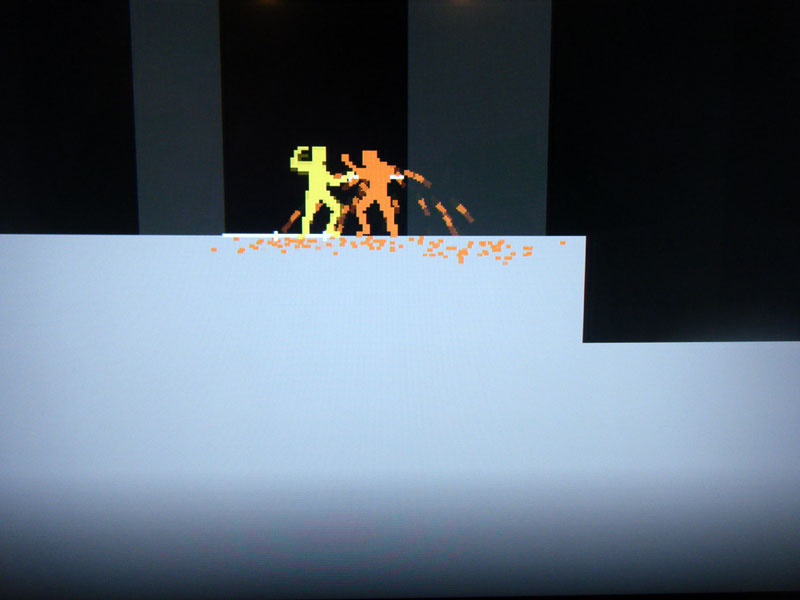This image from my computer game showcases a vividly colorful, landscape-oriented screen. The bottom of the screen features a dark bluish-gray hue that gradually transitions into a lighter blue shade as you move upward. The central focus is a platform on which two robot-like contestants are engaged in battle. The platform itself is a flat surface that steps down slightly, continuing as another flat blue plane.

On the left side, a yellow robot stands ready, while on the right, an orange robot faces it. The intense combat between the two results in orange specks scattering down onto the blue platform below. In the background is a black and gray striped area that adds to the scene's dynamic tension. Notably, both robots have small white sections in the middle, which appear to be the weapons they are using in their battle. The combination of vibrant colors, dynamic elements, and detailed background creates an engaging and immersive visual experience.